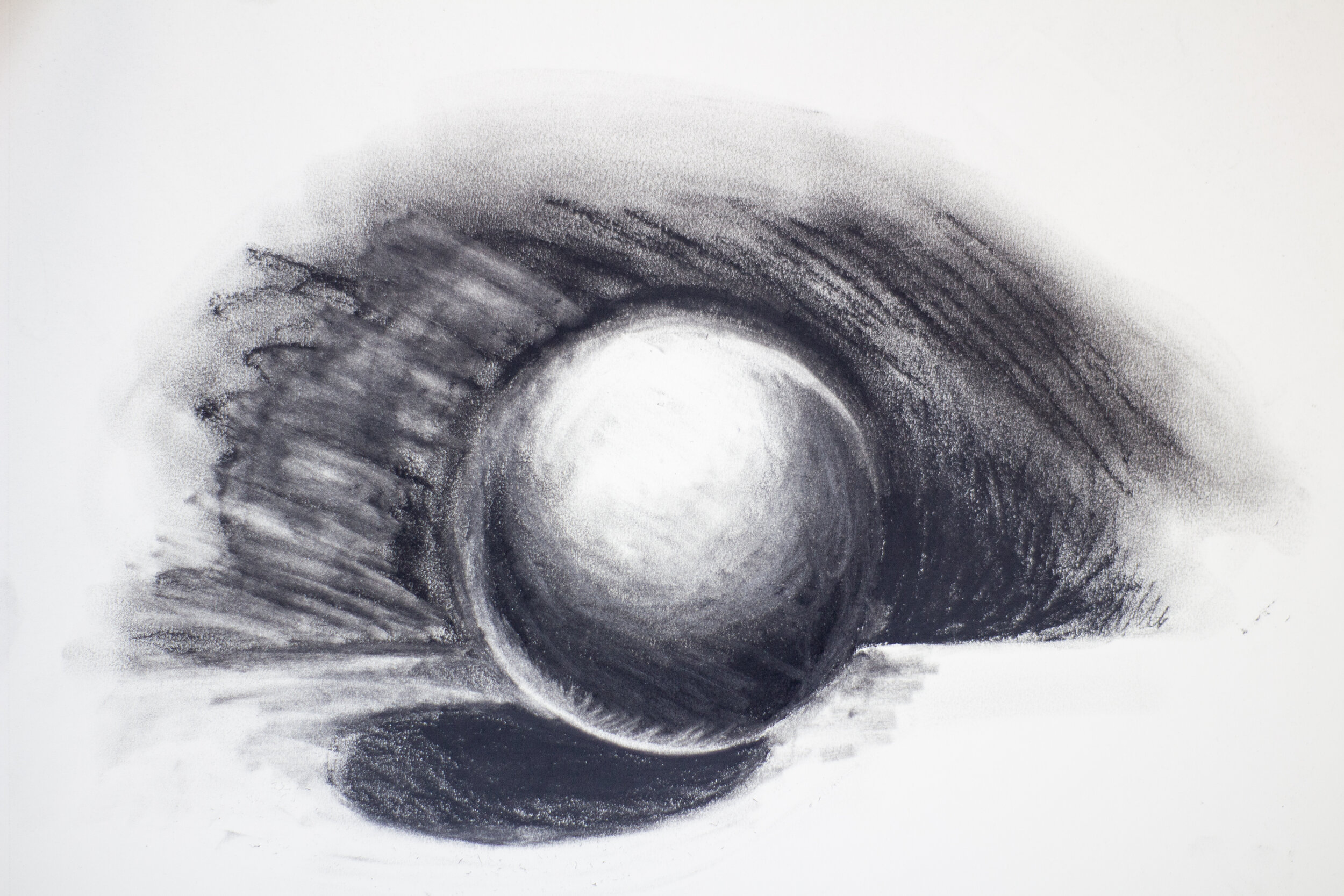In this detailed pencil drawing on simple white paper, an abstract and monochromatic scene unfolds. The central focus is a spherical object positioned in the middle of the image, reminiscent of a marble or possibly an eye that has emerged from its socket. This central sphere is outlined in black on the top and transitions to shades of white at the bottom, creating a gradient effect. The sphere casts a significant, dark shadow underneath it towards the bottom left, enhancing the depth and dimensionality of the artwork. Surrounding this main object are varying degrees of shadowing - with darker blacks on the right-hand side and a blend of black and white shadowing on the left. These shadows contribute to the abstract nature of the drawing, with the remaining areas filled with a grayish-white emptiness, giving the entire composition a stark and contemplative feel. The detailed shading and nuanced shadow work hint at meticulous craftsmanship, suggesting a sophisticated exploration of light and dark.